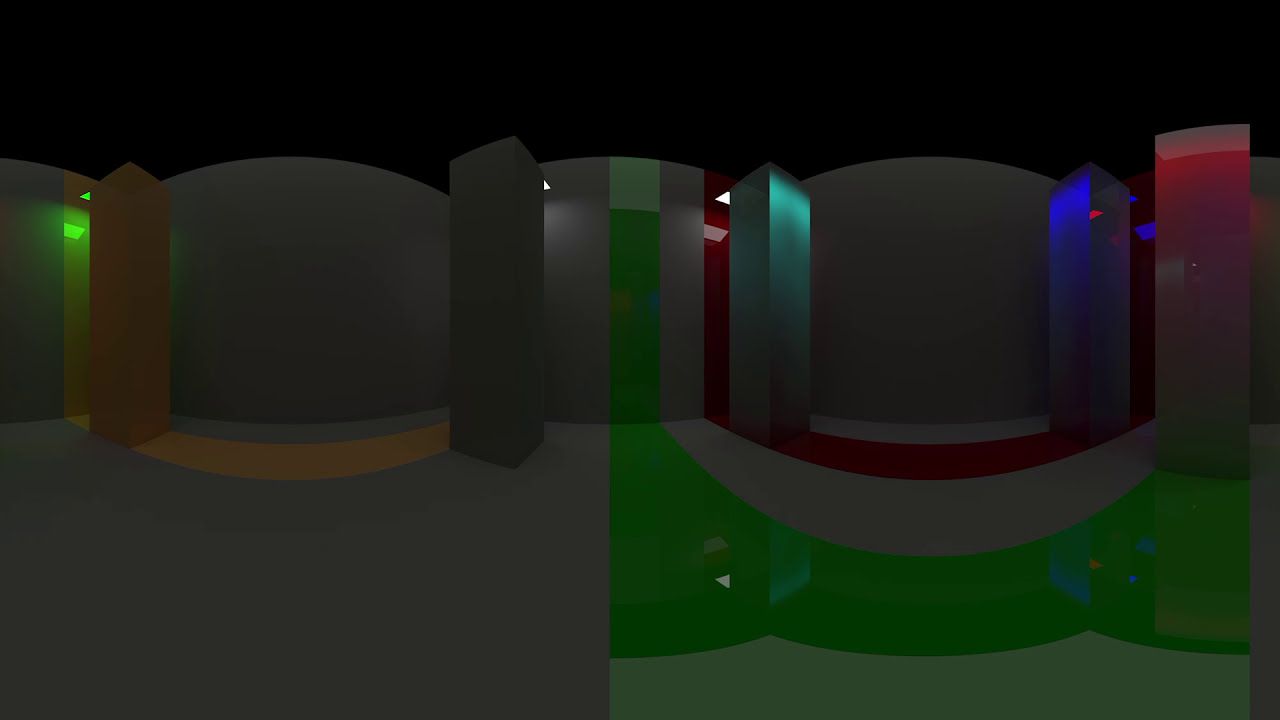The image is a complex, computer-generated 3D rendering of an abstract, fisheye perspective room with colorful lighting and reflections. Predominantly green, it features a wavy green stripe prominently in the lower right foreground, extending upwards and interacting with various elements within the scene. In the background, there is a red wall, creating a stark contrast. Adjacent to it, separated by a narrow gap, is a gray wall framed by blue and green pillars, each with a reflective quality causing them to catch hues of red, blue, and cyan light. The room also contains repetitive gray and brown pillars, adding to the multifaceted texture of the space. Despite the clear structure, the room lacks discernible objects, resulting in an abstract and somewhat indecipherable appearance, characterized by its rich colors and the interplay of light and shadow.